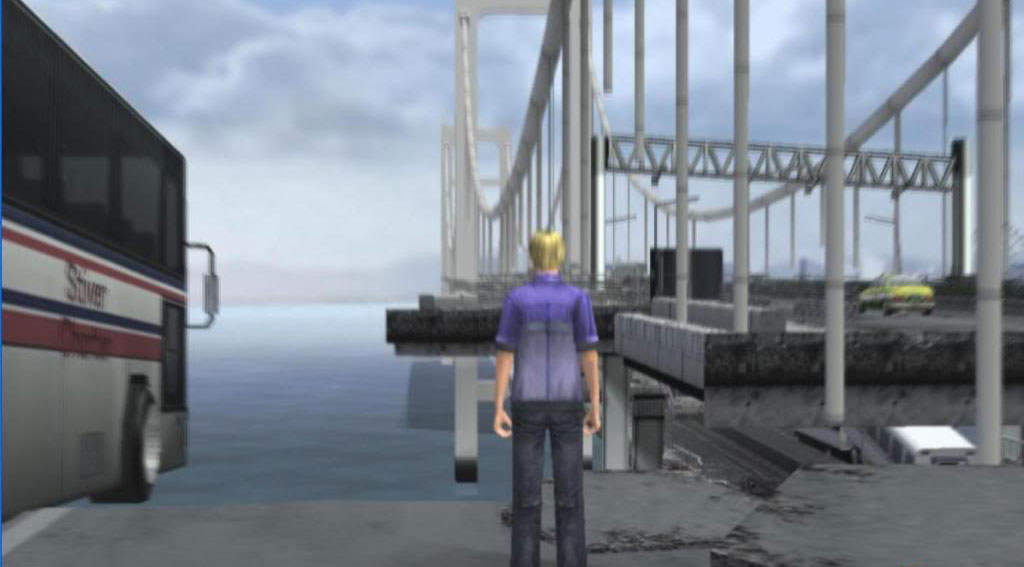In this outdoor photograph, the backdrop features a serene landscape characterized by a vivid blue sky adorned with scattered clouds. A thick layer of fog envelops the distant hills and sparsely dotted trees, creating a mysterious and tranquil ambiance. In the foreground, a large body of water, possibly the ocean, stretches out with gentle waves. Parked near the water's edge is a sizable bus with a striking design. The bus has a sleek black top and matching tinted windows. Its silver exterior is accentuated with bold red and blue stripes, along with prominent red lettering. Notably, a large handle extends from its door, adding to its imposing presence.

Adjacent to the bus, an impressive metallic silver bridge spans the water. Atop the bridge, a solitary yellow car traverses, adding a pop of color to the scene. In the foreground, a man stands in front of the bridge, clad in a short-sleeved blue shirt and dark trousers, gazing thoughtfully toward the horizon. This detailed and dynamic composition captures the essence of a peaceful yet vibrant moment in a picturesque outdoor setting.